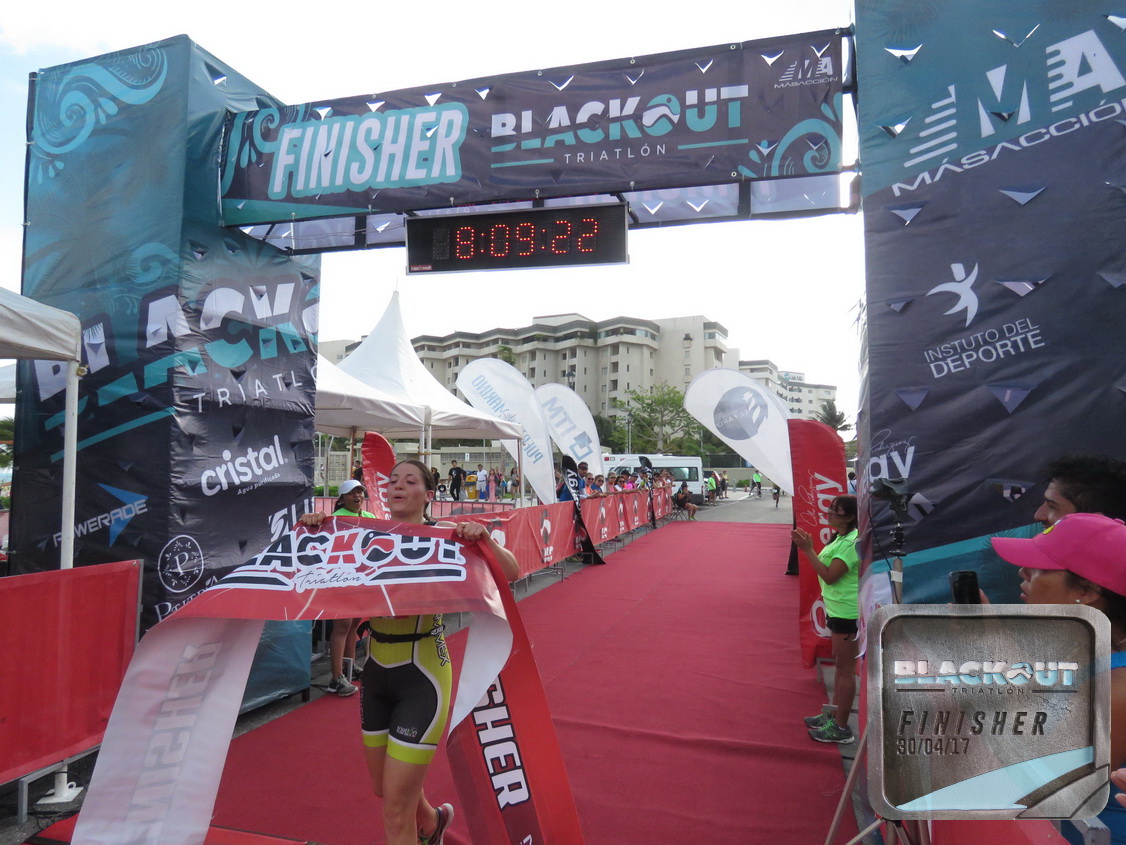The photograph captures the finish line of the Blackout Triathlon, prominently featuring a large archway adorned with black, blue, and green motifs. The archway bears the text "FINISHER BLACKOUT TRIATHLON" atop, along with a digital clock displaying a time of 8:09:22. Below the clock, a young woman in her 20s, clad in a black and yellow spandex suit, is seen triumphantly holding the finish line tape, indicating her position as the first to cross. The tape, emblazoned with "BLACKOUT" in red, black, and white, is stretched across a red-carpeted pathway. Throughout the scene, spectators are visible, clapping and cheering, some capturing the moment on their cameras. In the background, tall buildings, likely condominiums or apartments, stand as a distant backdrop. A silver block in the bottom right corner of the image displays “BLACKOUT TRIATHLON FINISHER 30.04.17.”